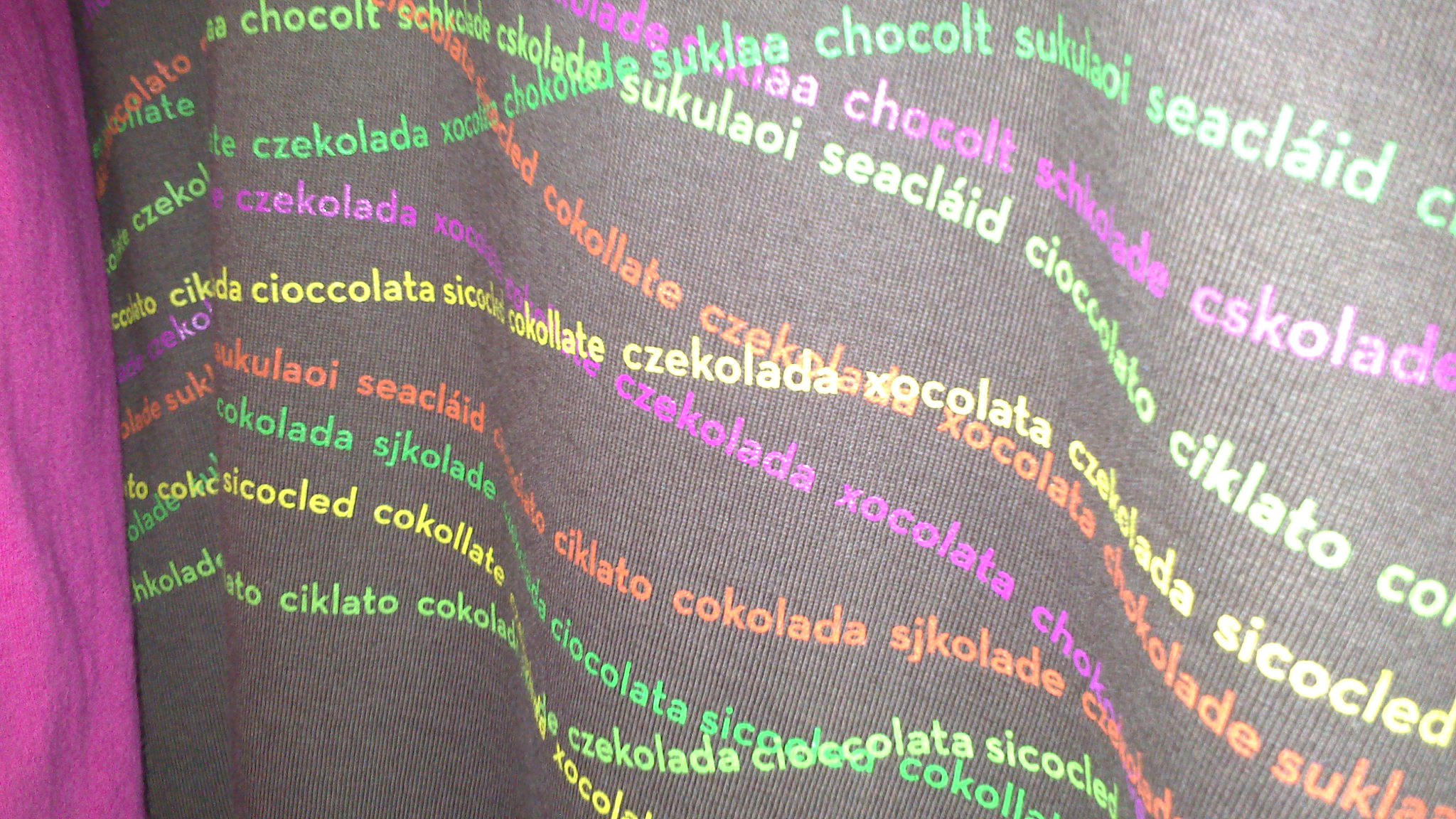This color photograph features three distinct blankets: a pink one on the far left, a smaller black one in the middle, and a larger brown blanket to the right. Both the black and brown blankets are adorned with text in an array of bright, neon hues including white, orange, neon green, neon yellow, and vivid pink. The text, not in English but in various other languages, appears to include the word 'chocolate' in multiple spellings, such as 'Chocolat' and 'Cioccolata', with words forming wavy, zigzagging patterns across the fabric, almost resembling colorful stripes. The vibrant words stand out prominently against the dark and brown backgrounds, adding a striking, lively visual element to the fabric.